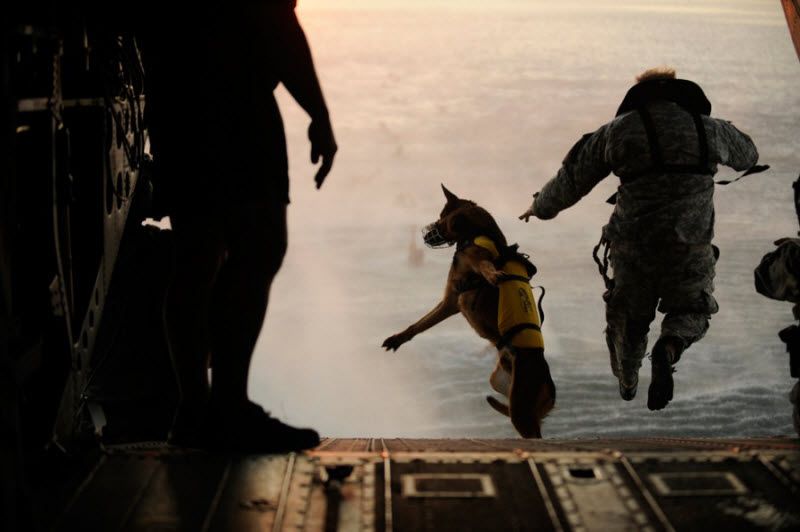In the dimly lit photograph, a German Shepherd dog and two soldiers are seen leaping out of a military aircraft, likely an army helicopter or plane, into turbulent ocean waters below. The platform beneath them features metal grates, characteristic of aircraft interiors. On the left edge of the open doorway, a male soldier stands watching the duo, his form partially silhouetted. Mid-air between the aircraft and the rough sea, the German Shepherd, equipped with a yellow life jacket, also appears to have a muzzle, jumps alongside the soldier dressed in a heavy green camouflage uniform and carrying a large backpack probably containing a parachute. The overall scene is dark, with the primary light illuminating the action being the open doorway, casting shadows and enhancing the drama of their daring dive.